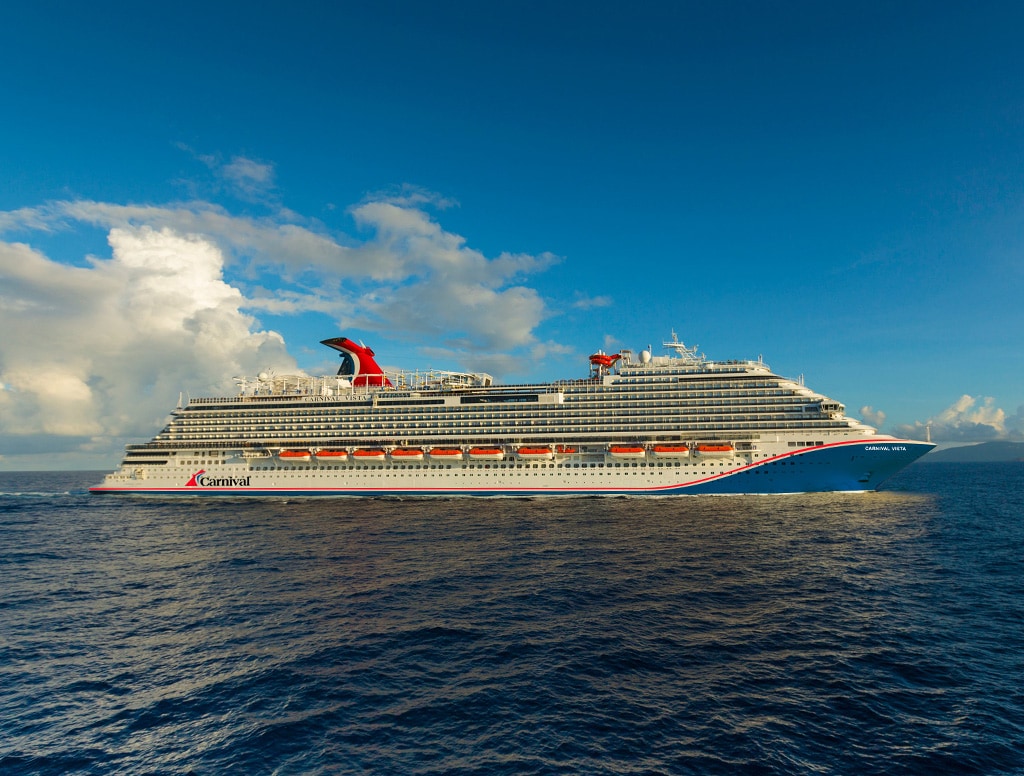The photograph captures the Carnival Vista cruise ship from a distance, positioned in a calm, dark blue sea. The ship is moving from left to right, its bow pointing rightward and its stern leftward. The main body of the vessel is predominantly white with a distinguishing blue swash under the bow and a red stripe running along its side. Visible towards the rear, the words "Carnival" label the ship. Multiple decks are stacked atop one another, each adorned with rows of tiny windows and portholes. Red and white lifeboats are attached along the ship's side beneath these windows. Above, the sky spans over half of the image, displaying a gradient from dark blue at the top to lighter hues near the horizon, interspersed with various low white and light gray clouds. A large hilly landmass appears in the distance on the right side of the image. The photograph, possibly taken by a drone or from a vantage point far enough and high enough to give a clear, detailed view, exemplifies representational realism.